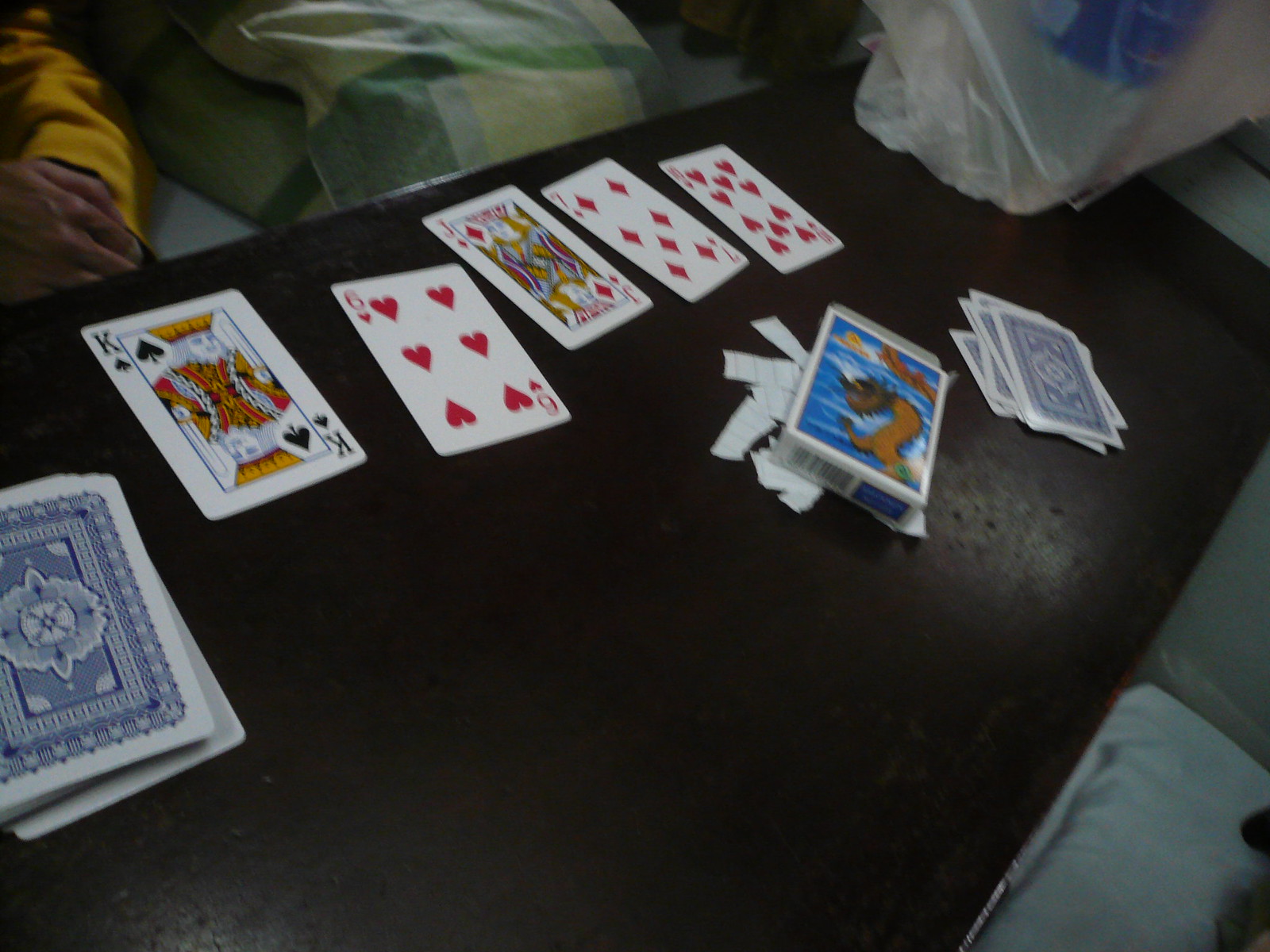The image captures a scene of a table, likely set on or near a couch as evidenced by the visible soft cushions framing the corners of the picture. On the table, a few cards are spread out alongside a larger stack of cards placed face down, suggesting a draw pile. To the right of this stack is a slightly smaller deck. Additionally, near these stacks is an opened pack that appears to have contained the cards, with paper strips scattered beneath it. The deck's box displays an image that looks like an ocean scene, possibly featuring a sea serpent or dragon. Displayed on the table face up are several cards held by someone's hand: a King of Spades, a Six of Hearts, a Jack of Diamonds, a Seven of Diamonds, and a Ten of Hearts. To the right, a plastic bag containing what seems to be an empty or partially filled drink bottle is visible, hinting that the person may have recently visited a store.